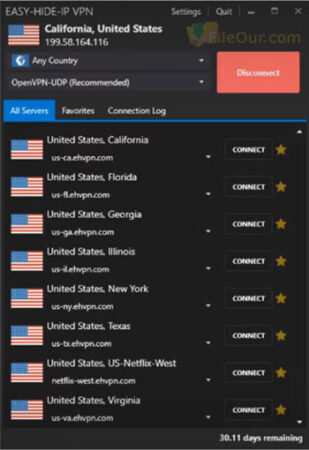This is a detailed screenshot of a smartphone displaying a VPN application with a dark or black theme. At the top of the screen, the app's name "EASY.HIDE.IPVPN" is prominently displayed in uppercase letters. On the right side of the top bar, there are options to access settings and quit the application.

Just below the top bar, there is a horizontal section featuring various interactive elements. On the left, an icon of the American flag is displayed next to the text "California, United States," followed by the IP address "199.58.164.166." To the right, there is a drop-down menu labeled "Any Country," as well as another drop-down menu specifying the VPN protocol as "OpenVPN.UDP (Recommended)." A red "Disconnect" button is also present in this section.

Further down, the interface provides navigation tabs with options for "All Servers," "Favorites," and "Connection Log." The current view is set to "All Servers."

Below the tabs is a list of VPN server entries, each marked numerically from 1 to 8, all featuring U.S. flags to the left of their respective entries. Each server entry provides the location and includes an interactive drop-down arrow and a "Connect" button to the right. The listed servers are as follows:
1. United States, California
2. United States, Florida
3. United States, Georgia
4. United States, Illinois
5. United States, New York
6. United States, Texas
7. United States, U.S. Netflix West
8. United States, Virginia

Additionally, all server entries have gold star icons next to them, indicating that they may be marked as favorites.